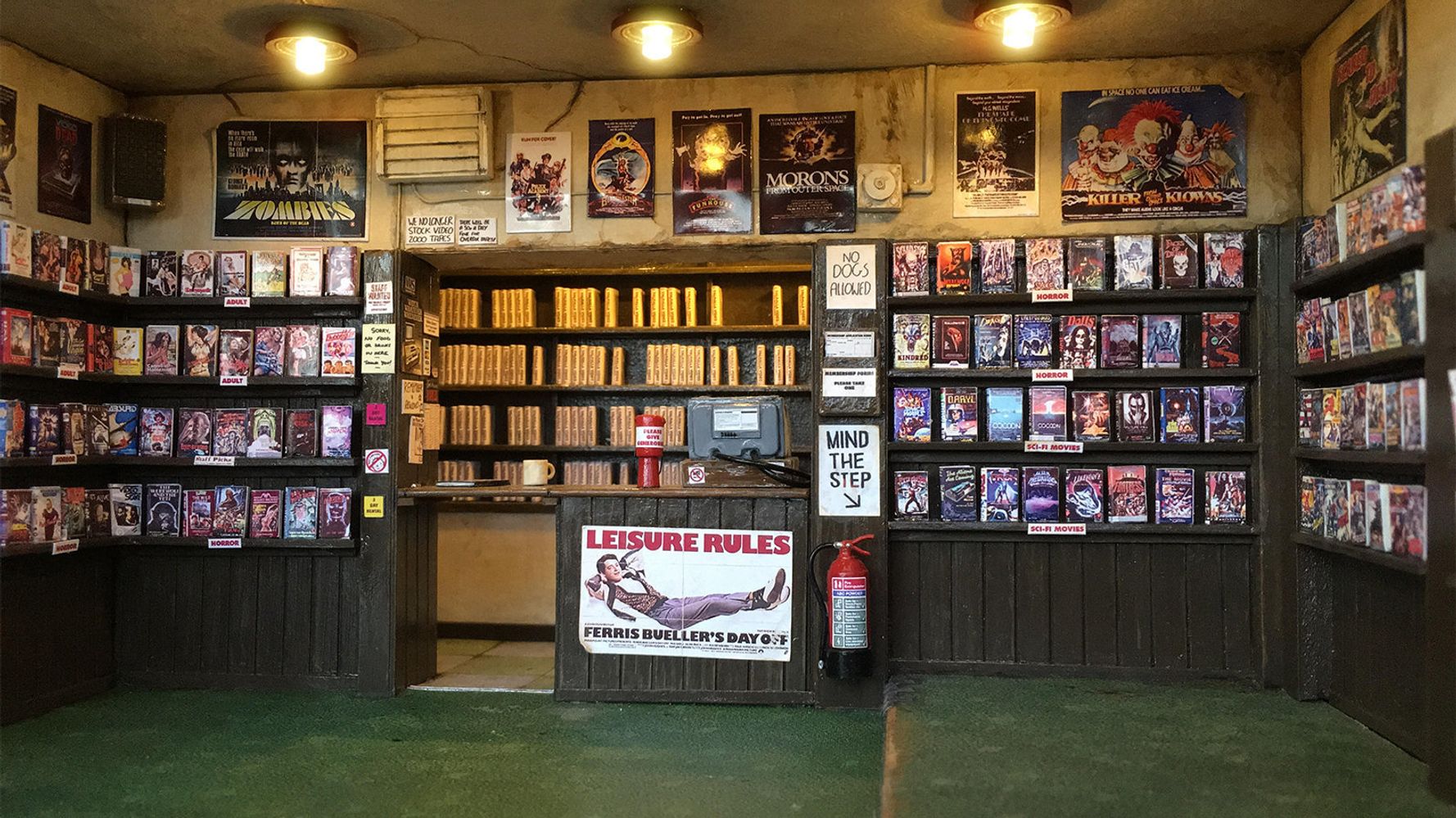The photograph captures the nostalgic essence of a small town, old-fashioned VHS rental store. The store features green flooring and wooden shelving lined with VHS tapes, primarily catering to horror and sci-fi genres along with a visible adult section. The top of the walls is adorned with various posters of 80s films, including ones featuring themes of zombies and killer clowns from outer space. The ceiling is equipped with three lights spaced evenly across. 

Near the entrance stands a makeshift counter with a sign prominently displaying "Leisure Rules, Ferris Bueller's Day Off." The counter holds an old-looking computer, a coffee cup, and a charity box, while signs like "Mind the Step" and "No Dogs Allowed" (both handwritten) are visible. A red fire extinguisher is placed beside the counter. The overall feel is slightly unkempt, emphasized by off-color white at the top of the walls, adding to the retro ambiance of the cherished video rental spot.